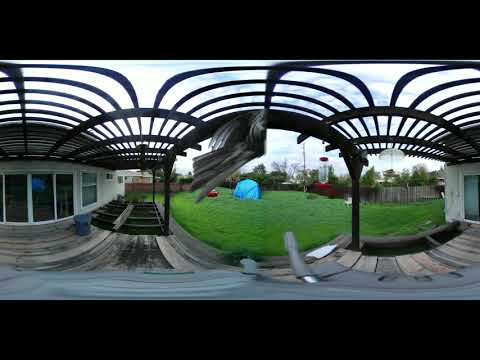The image captures a unique backyard view of a house with a mirrored yet distinct appearance on each side. The house features a rounded design and is painted white, with a row of rectangular windows on the left section. There's a wooden porch in front, extending into a walkway, alongside a wooden archway or gazebo-like structure with thin, open-ended, black architectural elements resembling large hand fans, five in total. The middle of the scene is open, revealing bright green, well-trimmed grass that sprawls from the mid-left to the far right, partially hiding a wooden fence and some bushes. In the center of the lawn sits a large, blue tent or tarp-like item. Nearby, a red hummingbird feeder with a clear glass jar stands out against the greenery. The right side of the image shows another section of the house with a rectangular opening or window, lightly tinged blue. The background includes some trees under a slightly cloudy sky, contributing to the serene ambiance. Towards the bottom of the image, close to the camera, a gray pavement, possibly a driveway, is visible.